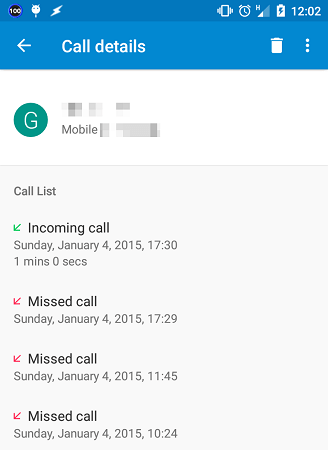This is a vertically oriented image captured from a smartphone screen. The background exhibits a subtle transition, possibly due to the display settings, ranging from a yellowish beige to a light blue shade. At the top, it features two shades of blue: a darker blue strip across the top followed by a slightly lighter blue beneath it, yet both are within the darker spectrum of blue hues.

On the upper left side of the screen, several icons are visible, including a lightning bolt icon, a "100" within a black circle, and another charging-related symbol. The upper right corner displays the current time (12:02) alongside icons for battery status, Wi-Fi, and signal strength.

In the lighter blue section below, there are navigational elements including a back arrow, a call detail icon, a trash can icon on the right side, and three vertical dots indicating more options.

Further down in the white section of the screen, there's a recognizable green circle with a white "G" in it. The content here is somewhat blurred, but it is clear enough to identify certain details. The title "Call List" and "Incoming Call" are visible along with the specifics of a call made on Sunday, January 4th, 2015 at 17:30 (military time), lasting 1 minute and 0 seconds. Additionally, there are three missed calls listed with red arrows pointing downward, indicating the times and dates: one at 17:29, another at 11:45, and the last at 10:24, all on the same day, January 4th, 2015.